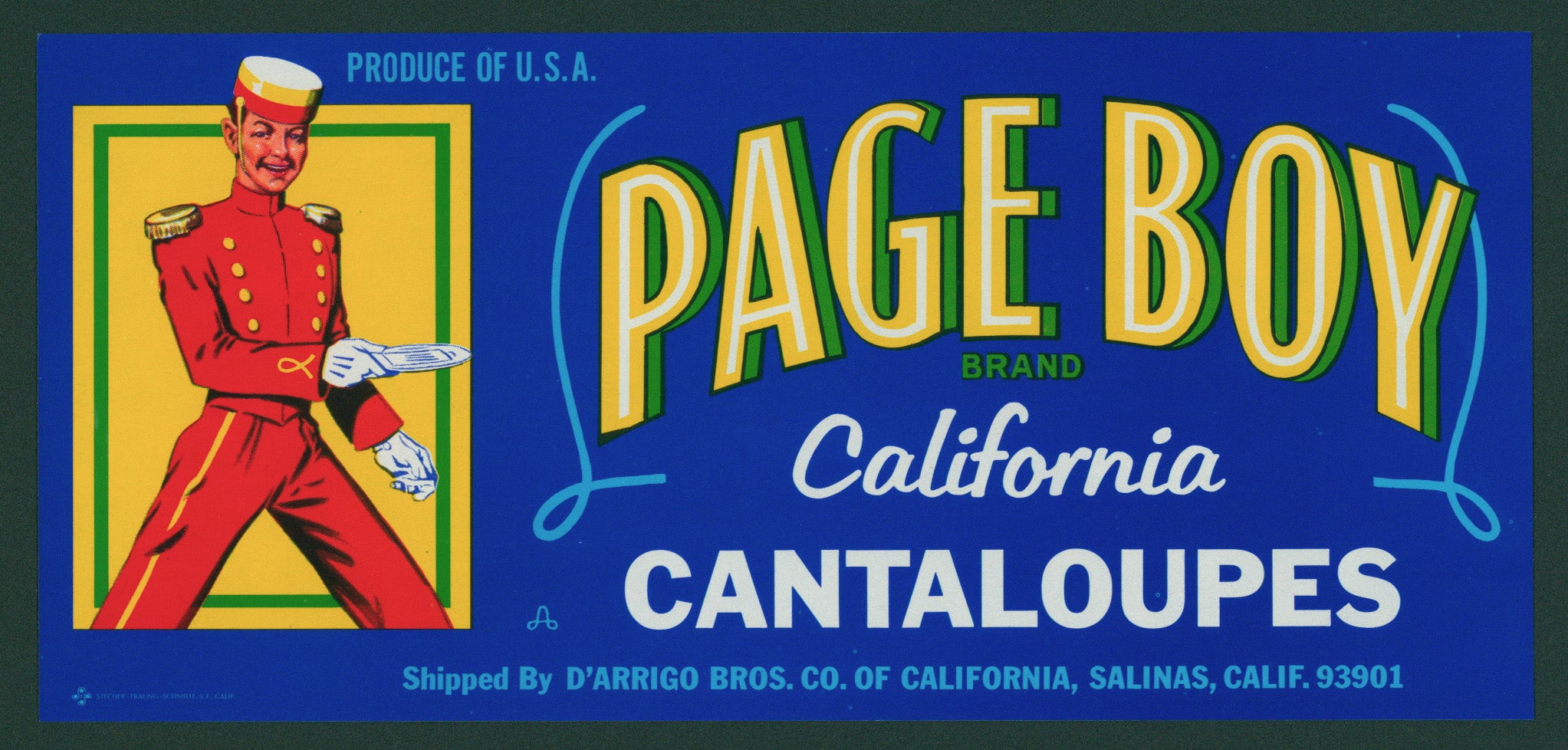This image depicts a vintage advertisement for Pageboy brand California cantaloupes. The advertisement features a striking royal blue background framed by a quarter-inch thick black border. Positioned in the upper left corner are the words "Produce of USA." Below this text is a notable graphic element: a yellow square encasing a green block that prominently displays a bellboy figure. The bellboy, presumably representing the "Pageboy" brand, is dressed in a distinctive red suit adorned with gold shoulder epaulettes, gold ribbon details, golden buttons, and white gloves. He wears a red, gold, and white hat, exuding an old-world charm reminiscent of a hotel usher or marching band leader. 

The brand name "Pageboy" is prominently displayed in block letters with a bold green shadow and a gold front, further highlighted by white detailing. Below this, "California" and "Cantaloupes" are written in clear white text. At the bottom of the advertisement, in a lighter blue text, it reads, "Shipped by the D’Arrigo Brothers Company of California, Salinas, California 93901." The cohesive design and vibrant colors give this advertisement a classic and timeless appeal.